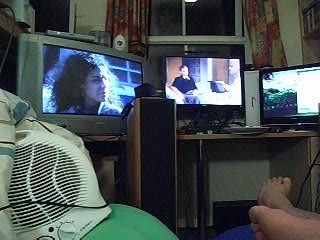The photograph depicts a cozy living room scene, with a central focus on a window adorned with multicolored curtains, indicating it might be nighttime outside. In front of the window, two tables support three different screens. On the left, an older silver television displays an image of a woman with brown, frizzy hair looking over her left shoulder. The central screen, which appears to be a television, shows a man in a black shirt sitting on a white couch, seemingly resting his hand under his chin. To its right stands a computer monitor showcasing a scenic view of green mountains, possibly accompanied by a small window with additional content. 

At the bottom left corner of the image, a small white fan sits atop a round, green object, which might be a blanket. Meanwhile, the bottom right-hand corner reveals a pair of feet, suggesting the photo is taken from the perspective of someone lounging with their legs outstretched, potentially on a bed or sofa. This intimate snapshot provides a glimpse into a relaxed private space, filled with diverse visual entertainment and a sense of calm.